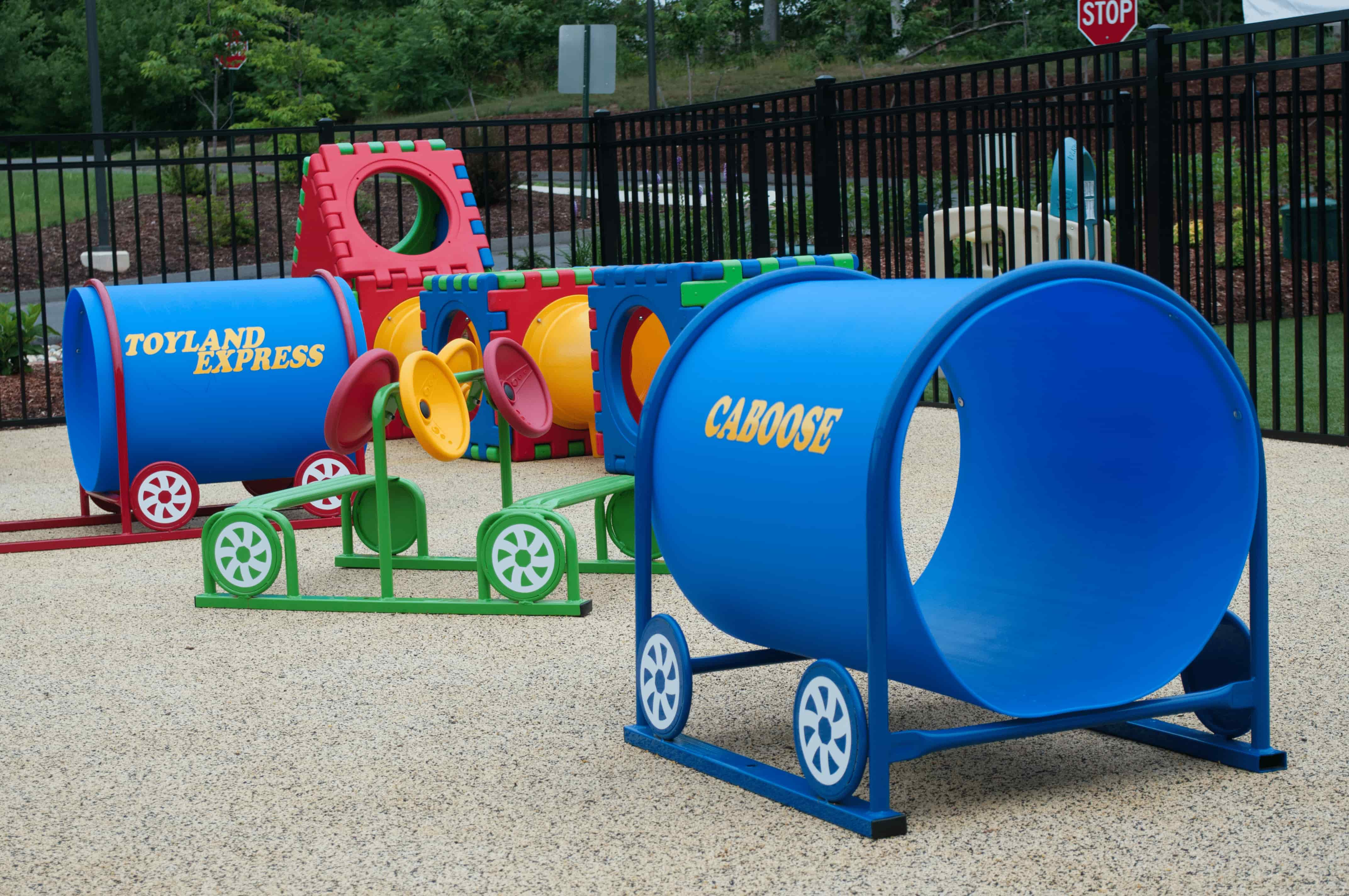The photograph depicts a children's playground enclosed by a black railed fence, situated within a park-like area featuring trees, grassy hills, and two visible stop signs lining a road in the background. The main play structures are designed to resemble a train, with large blue cylindrical tubes adorned with bright yellow text. One tube prominently reads "Toyland Express" and is equipped with decorative red wheels, while another labeled "Caboose" features blue wheels. The play area includes additional playground elements such as benches with green circular discs and plastic tunnels for crawling. The ground itself appears to be covered in a soft, speckled material, enhancing the play area’s safety.